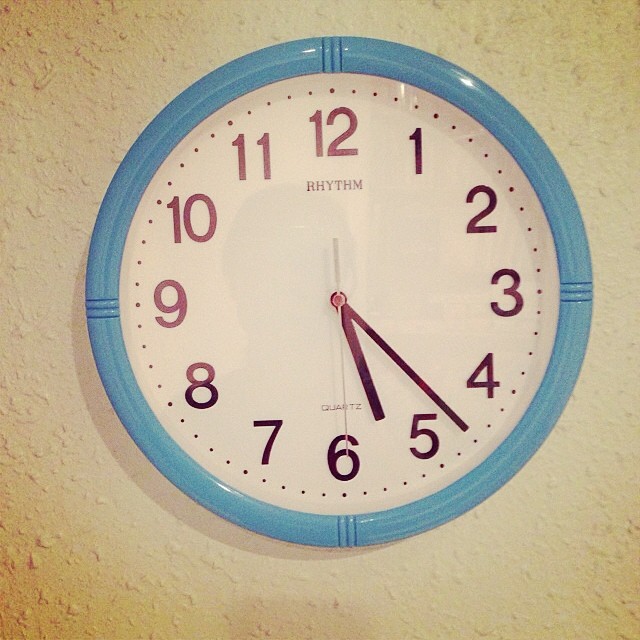This image showcases a circular blue wall clock with a sleek design. The clock’s face is white, providing a clear background for the black hour numbers, ranging from 1 to 12, which are evenly spaced around the dial. Prominently, the clock features a trio of blue lines extending outward from its edge at the 3, 6, 9, and 12 o'clock positions, adding a decorative yet symmetrical touch.

The clock is equipped with three hands: an hour hand, a minute hand, and a second hand. At the time the photo was taken, the time displayed is approximately 5:23. A notable detail in the image is the way light falls on the clock, casting a subtle brown hue over the numbers 8, 9, 10, 11, and 12, creating an interplay of shadow and light. This visual effect adds a unique characteristic to the otherwise simple and functional timepiece.